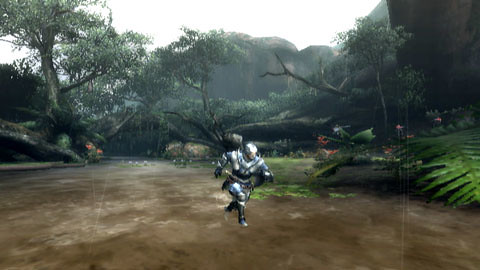The image is a screenshot from a video game featuring a knight in motion. The knight, clad in full silver armor with a blue tunic underneath and black gloves, is captured in mid-stride, running along a dirt path. His armor includes a helm, chest armor, shoulder armor, gauntlets, leg plates, and greaves. Equipped with a war maul or war hammer, the knight is moving towards the camera's point of view. The environment is rich in detail: on the left side, there are large trees with red flowers at their base, while the right side shows green plants and large green leaves. The central and bottom parts of the image display a muddy brown and tan path, interspersed with patches of green grass. The backdrop features mountains or hills under a clear sky, adding depth to the scene.